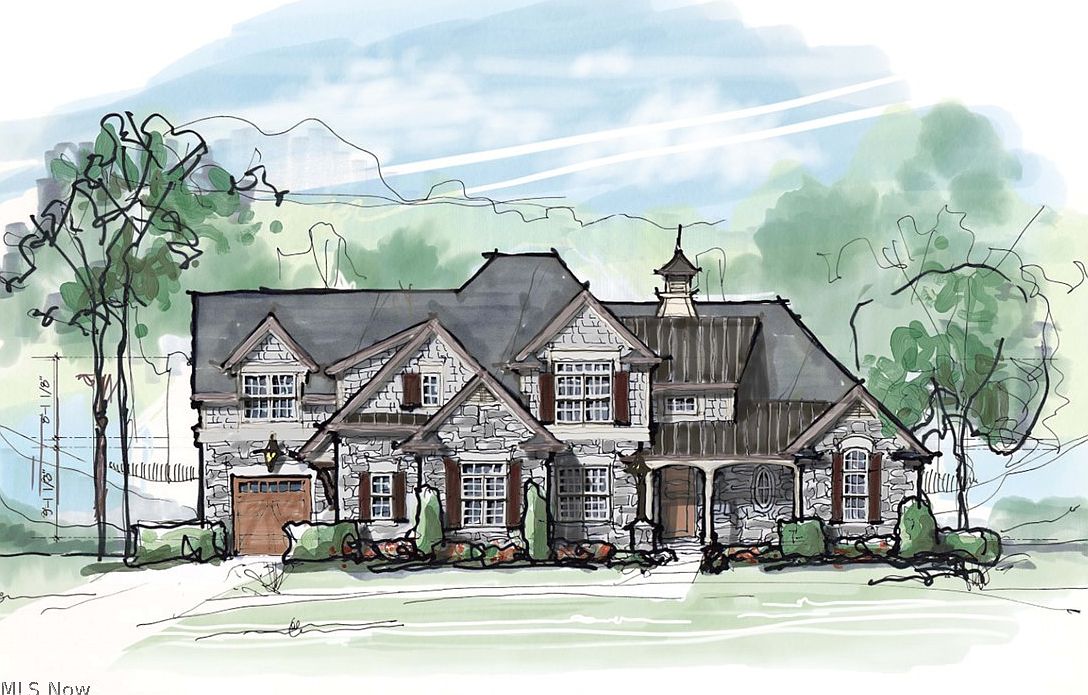The image depicts a detailed and beautifully crafted ink and watercolor artwork of a large mid-century style house. The house, primarily sketched in black ink, incorporates a mix of grayscale bricks with hints of pastel green, offering a unique, artistic flair. Prominent columns flank the main doorway, while a red-hued garage door sits at the extreme left. The structure boasts multiple stories and an assortment of windows, some larger and some smaller, accented with dark brown window covers. The gray roof and two smaller additional roofs contribute to the house's grand appearance, featuring a chimney that extends slightly above the roofline. The lawn and decorative plants, all painted in pastel green, blend harmoniously with the two flanking trees on either side of the house and additional trees in the background. A well-defined pathway leads from the driveway to the brown front door. The artwork exudes a serene rural vibe, further accentuated by horizontal green shading to represent grass beneath the house. In the bottom left-hand corner, there is a subtle inscription that reads "MLS, Now."